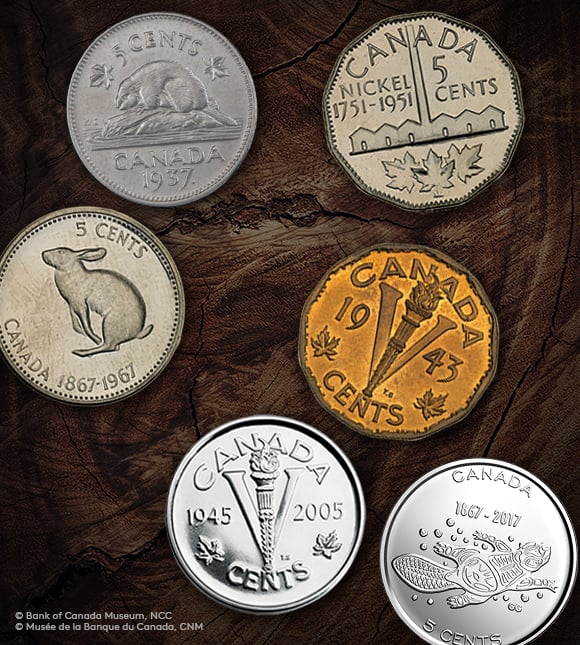This is a close-up photograph of six different Canadian 5-cent coins laid flat on a dark wooden surface, all featuring distinct historical designs. In the top left, a silver coin displays a beaver sitting on a log with the inscription "Canada 1937." To the right of this is a coin with an irregular, edged shape that reads "Canada nickel 1751 to 1951, 5 cents," showcasing buildings with a prominent central tower above three maple leaves. Below to the left, another round silver coin is engraved with "Canada 1867 to 1967" and depicts a jumping rabbit or hare. Adjacent to it is a silver coin marked "Canada 1945 to 2005" with a V and a torch at its center. Positioned above this, a brass-colored coin features the same V and torch motif with the inscription "1943." In the bottom right, another silver 5-cent piece displays "Canada 1867 to 2017" with an abstract representation of a beaver, appearing almost skeletal, against a smooth background. All coins rest on a dark wooden surface, with a copyright marking from the Bank of Canada Museum visible in the lower portion of the image.